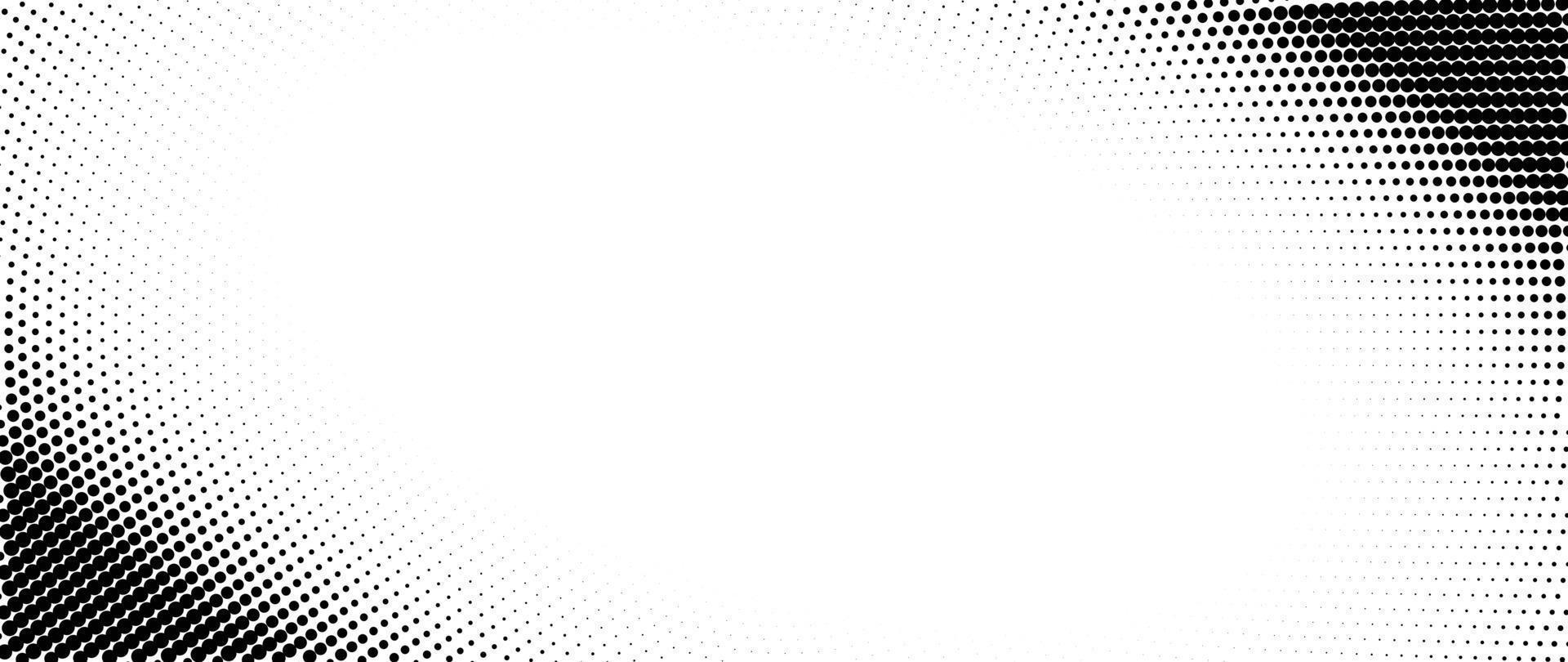The image resembles a pop art piece depicted in black and white. It is a horizontally oriented rectangle. Dominating the center is an oval shape, placed diagonally from the bottom left to the top right, which is strikingly bright white. Radiating from the central oval, the image features numerous black dots that start small near the white center and progressively grow larger and denser towards the top right and bottom left corners. This gradient creates a cloudy, out-of-focus effect around the edges, fading to gray in the top left and bottom right corners. The overall composition gives the illusion of looking into a curvilinear, perforated tunnel, akin to the inner surface of a stainless steel dryer drum, emphasizing the dots' curved and immersive arrangement.